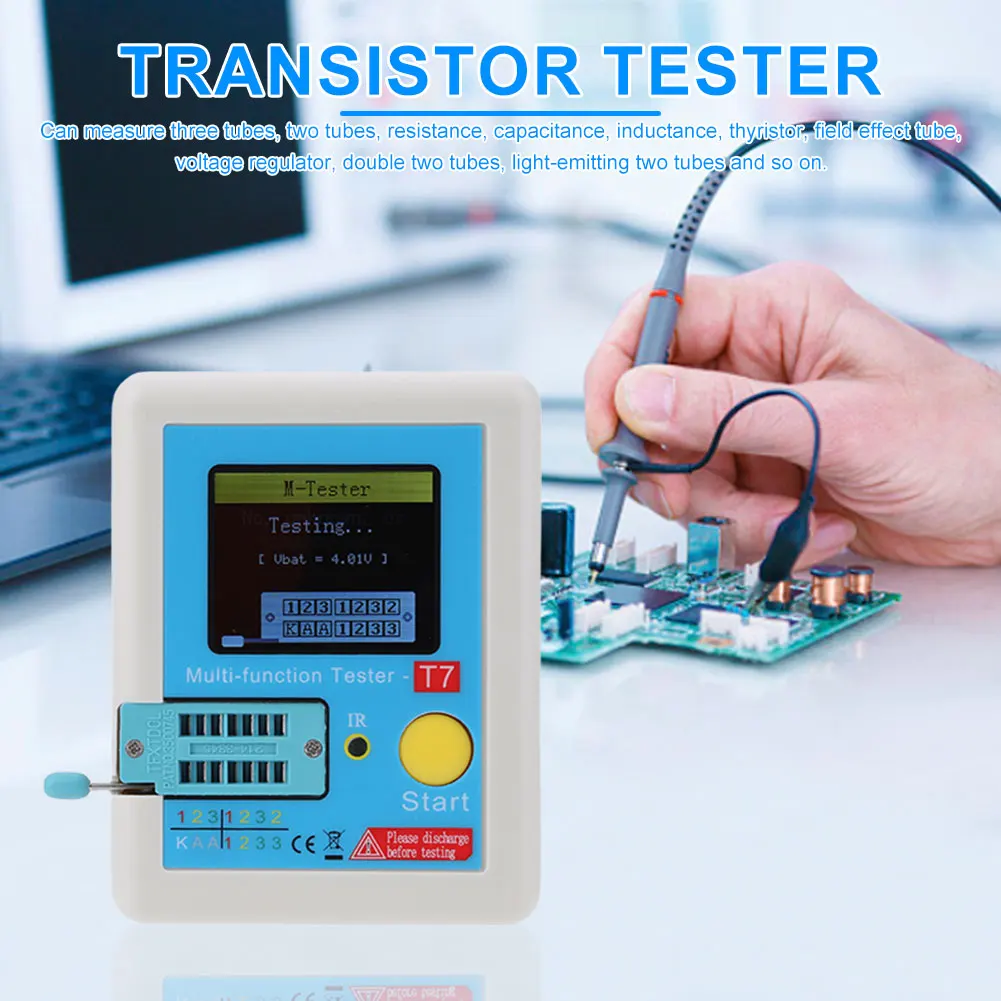The image showcases a perfectly square advertisement for a Transistor Tester. At the top, in prominent blue text outlined in white, are the words "Transistor Tester." Below this, separated by a blue horizontal line, is smaller blue text listing the device's capabilities: "can measure 3 tubes, 2 tubes, resistance, capacitance, inductance, thyristor, field effect tube, voltage regulator, double 2 tubes, light emitting 2 tubes, and so on." 

In the lower left-hand corner of the image is the device itself, featuring a white border surrounding a blue panel. The device is labeled "Multifunction Tester" and includes a screen displaying "M-Tester Testing, VBAT = 4.01V" with a slightly blue-hued readout showing numbers such as "1231232, KAA1233." Below this screen is a yellow button labeled "Start," and the panel houses several slots and a slide lever at the bottom left.

To the center right of the image, a Caucasian hand is seen holding a probe connected to a green circuit board with copper wires and other components. The background features a blurry depiction of what appears to be a computer screen and keyboard on the left and some additional electronic components. The entire advertisement is framed with a blurred white background, directing attention to the Transistor Tester and its functionalities.